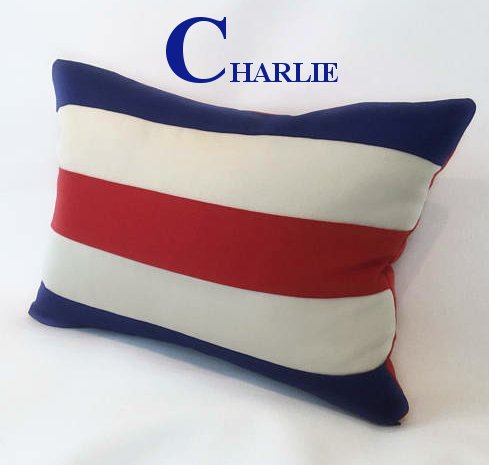The image features an overstuffed throw pillow prominently displayed against a bright white wall that extends to a floor, creating visible shadows around the pillow. The pillow showcases a pattern of five horizontal stripes in navy blue, off-white, red, off-white, and navy blue from top to bottom. The pillow's edges are outlined with red piping, suggesting that the backside of the pillow may be entirely red. Above the pillow, the word "CHARLIE" is displayed in all capital, serif-font blue letters, with the letter "C" noticeably larger and more elaborate than the rest. The font choice and the styling of the letters give a distinct impression, potentially indicating the name of the pillow or its brand.